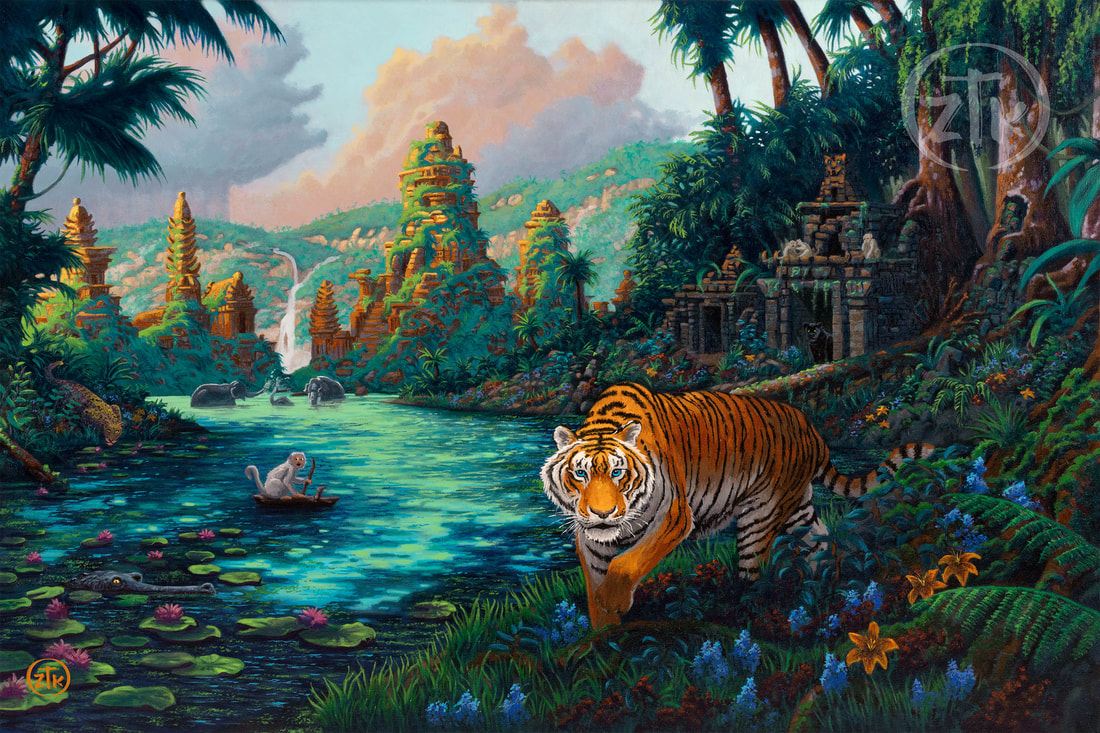This painting portrays a captivating jungle scene with a central focus on a fierce lion predominantly orange with black stripes, blue eyes, and white accents on its edge of the face and underbelly. The lion appears to be prowling with a forward gaze, and its front paws possibly lifted. Positioned on the riverbank, the lion is surrounded by a lush, tropical environment. The green river nearby is dotted with lily pads and pink flowers, and it contains a monkey steering a small, makeshift boat with a stick. 

Nearby, a green alligator with gold eyes lurks in the water. In the distance, the river hosts a family of three elephants—two adults flanking a child—creating a heartwarming scene. The right-hand side of the painting features a shoreline packed with verdant jungle vegetation and ancient Mayan temple ruins, now overgrown. The river itself is a bright, bluish turquoise, adding a sense of vibrancy to the setting, which is further enriched with various orange and blue flowers, large trees, ferns, and distant waterfalls cascading over rocky cliffs and hillsides, enhancing the painting’s enchanting and mystical atmosphere.